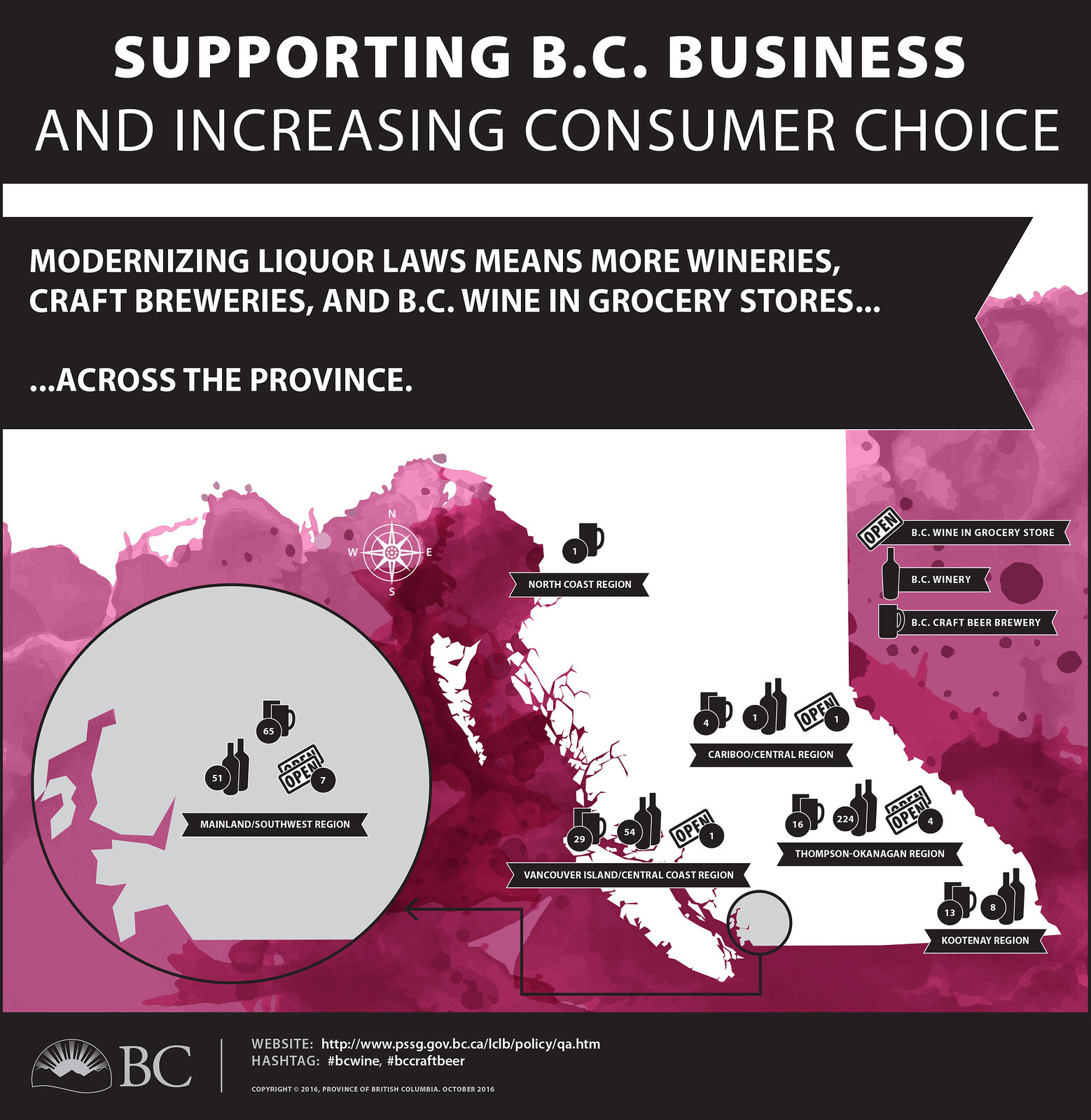The image is a detailed print advertisement set against a white background, primarily featuring a map with bright pink, rosy, and purply hues to highlight various regions in Vancouver, BC. At the top of the image, a black banner with white capital letters reads, "SUPPORTING BC BUSINESS AND INCREASING CONSUMER CHOICE." Below this, another black banner with slightly smaller white capital letters states, "MODERNIZING LIQUOR LAWS MEANS MORE WINERIES, CRAFT BREWERIES, AND BC WINE IN GROCERY STORES ACROSS THE PROVINCE."

The main central section showcases a purply-colored map divided into several labeled regions, each marked with relevant icons and numbers. For instance, the "Mainland/Southwest Region" features icons of two black wine bottles labeled '51', two beer mugs labeled '65', and two 'Open' signs marked '7'. A compass icon and a circle are also present within this region.

On the left side, an icon of a beer mug with '1' denotes the "North Coast Region". Over to the right side, the map indicates "BC Wine in Grocery Store" with an adjacent black silhouette bottle labeled 'BC Winery' and a beer mug icon for 'BC Craft Brewery'. The central portion of the map also highlights the "Cariboo Central Region" with icons: two beer mugs marked '4', two black bottles labeled '1', and an 'Open' sign marked '1'. Additionally, the "Vancouver Island Central Coast Region" lists 29 black mugs, 54 black wine bottles, and one 'Open' sign.

The "Thompson Okanagan Region" includes 16 black mugs, 224 black bottles, and four 'Open' signs. Lastly, the "Kootenay Region" at the bottom right corner of the map displays two mugs marked '13' and two bottles labeled '8'.

At the bottom of the image, another black banner features a logo with a sun design and the letters 'BC' next to it, along with a website URL providing further information.